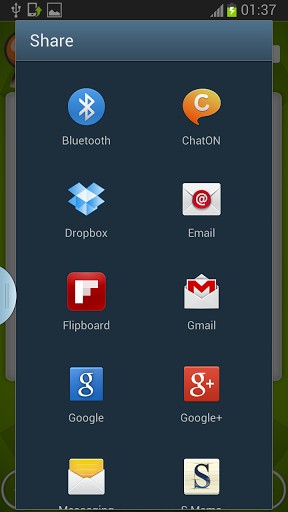The screenshot depicts a smartphone screen with a dark background. At the top right corner, the time is displayed as 1:37, although it is not specified whether it is a.m. or p.m. The battery icon is green with a small white lightning bolt, indicating that the phone is currently charging.

Dominating the screen is a large vertical rectangular pop-up box. The top border of the box is dark blue, with the word "Share" in white text on the left. Below this, the main portion of the box has a slightly darker blue background, featuring two rows of icons arranged in two columns.

In the left column, from top to bottom, the icons are as follows:
1. Bluetooth – represented by a blue circle.
2. Dropbox – symbolized by its iconic logo.
3. Flipboard – recognizable by its standard app icon.
4. Google – an old logo, approximately 10 years old, showing a light blue background with a small white letter "G."
5. Email – denoted by a traditional envelope icon.

In the right column, from top to bottom, the icons are:
1. ChatON – depicted as an orange bubble with a large white letter "C."
2. Email – indicated by a white envelope icon, identical to the one in the left column.
3. Gmail – represented by an older logo consisting of just a red "M."
4. Google+ – displayed as a light red background with a small white letter "G" and a white plus sign. It's worth noting that Google+ is no longer in existence.
5. An unidentified app – marked by a simple white square with the letter "S." The full name of the app is cut off at the bottom.

The overall design and app icons suggest the screenshot is from an older version of a smartphone operating system.